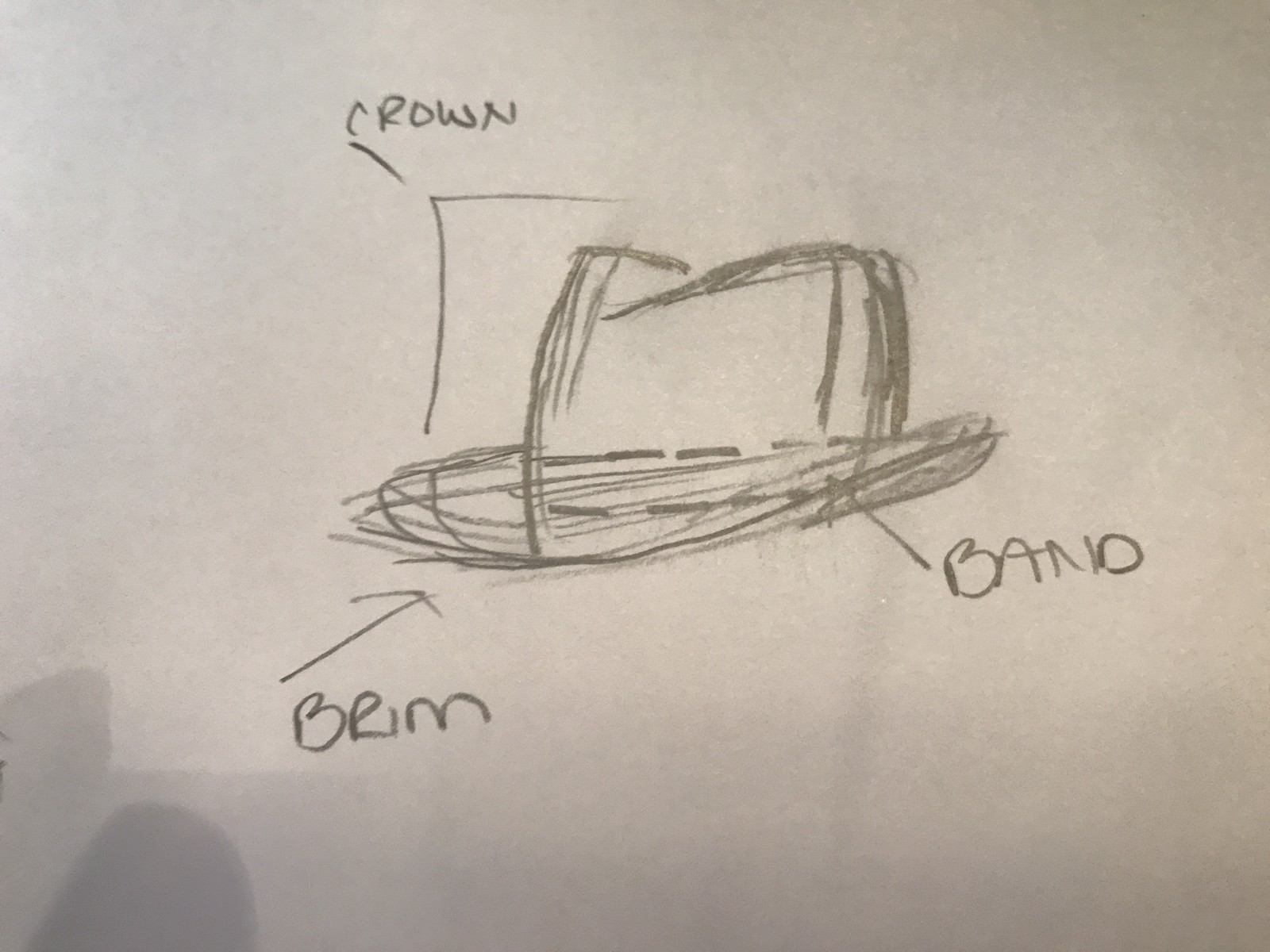This detailed blueprint showcases the preliminary design of a cowboy-style hat, meticulously hand-drawn in pencil. The sketch prominently features a large crown and rounded sides and front, characteristic of a traditional cowboy hat. Arrows extend from various parts of the hat to annotations specifying its key elements: the crown, brim, and band. Notably, the arrow pointing to the crown is split, indicating the encompassing range of the entire top section of the hat. The hand-drawn nature of this blueprint is evident through the numerous strokes and rough lines that outline and accentuate the hat's dimensions and features, embodying the initial stages of its design process.